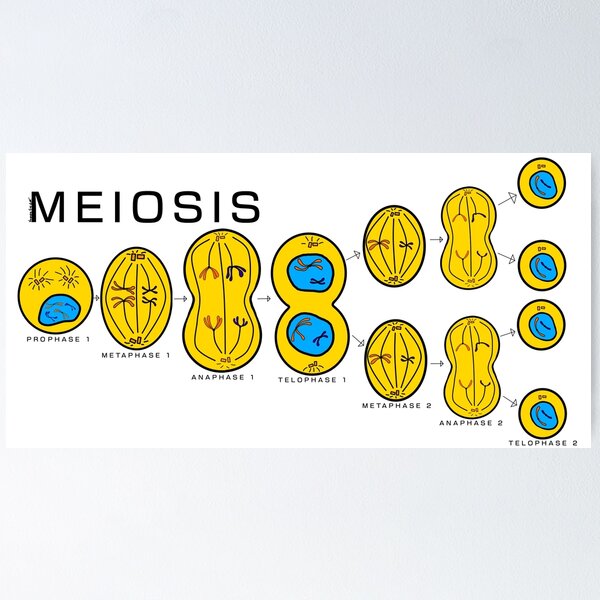This is a detailed scientific chart labeled "MEIOSIS" at the top left in black lettering on a white background. The chart visually breaks down the stages of meiosis, featuring illustrations in yellow and blue with black lines. Starting from the left, the diagram begins with a yellow circle containing a blue cell, labeled "PROPHASE 1." To its right is an elongated yellow oval captioned "METAPHASE 1." Moving further right, the diagram shows a larger figure-eight-like shape labeled "ANAPHASE 1." Next, to the right of "ANAPHASE 1," is an even larger figure-eight illustration with two blue cells in the middle, labeled "TELOPHASE 1."

From "TELOPHASE 1," the chart branches into two separate sequences. Each branch starts with "METAPHASE 2," followed by "ANAPHASE 2," and then splits into four separate illustrations labeled "TELOPHASE 2." The images grow larger through each phase, initially branching into two illustrations in "TELOPHASE 1" and ultimately splitting into four in "TELOPHASE 2." There is no additional explanatory text on the chart besides the labels of the phases.